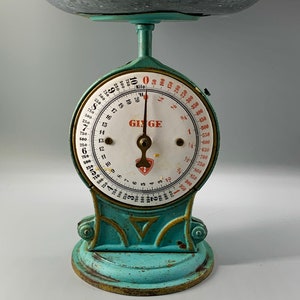This close-up color photograph captures a vintage analog scale, showcasing its ornate, patina-green base adorned with intricate curlicue designs. The scale, showcasing a robust turquoise hue with rust and wear indicative of its age, sits on a light gray table against a dark gray background. The circular dial in the center, framed by the faded paint and rust, has a distinctive design with a downward-facing triangle and curled metal frills on either side. The dial features numbers from 0 to 10, with the left half in red and the right half in black, and the needle points upwards at zero. An obscured word, possibly "GINGE," is partially hidden under the needle, accompanied by a red emblem resembling a Swiss cross. At the top of the frame, the lower part of the tray for weighing objects is just visible, supported by a dark blue-green stem. The scale exudes a shabby chic aesthetic, rich with character and historical charm.